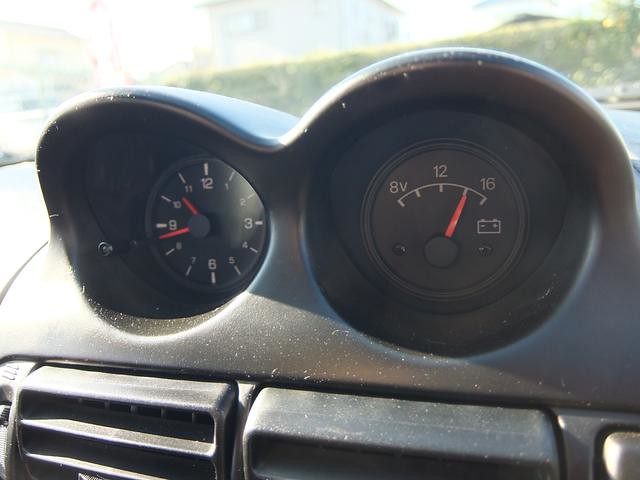The photo captures the interior of a car with either a deep brown or black dashboard. Prominently featured are two rounded humps on the dash, each housing an essential gauge. The right hump contains a battery gauge, detailed with a white line and a small black circular piece with a red pointer. This gauge displays readings of 8, 12, and 16 volts and includes a miniature battery icon marked with minus and plus symbols. The left hump features an elegant black clock with white markings and numbers, adorned with two vibrant orange hands indicating the time, set at approximately 10:43. Below these gauges are two air vents; the right vent is adjusted lower than the left one, indicating active airflow. This image offers a rich, close-up view of the intricate and functional elements of the car's dashboard.